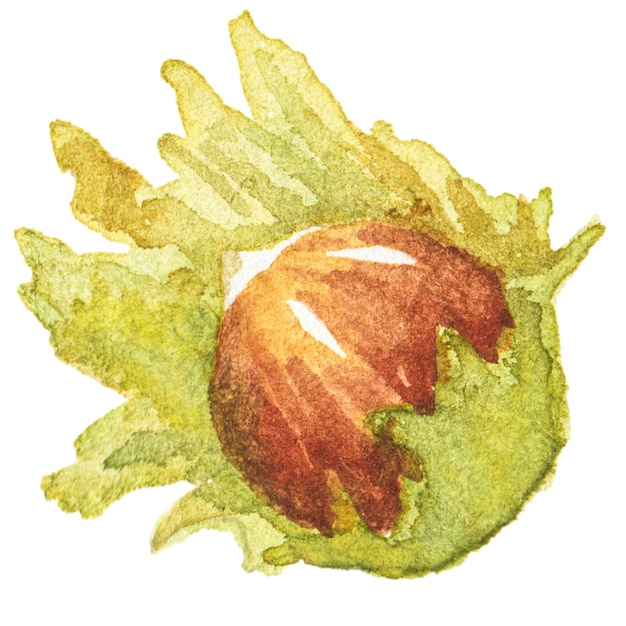The image depicts a detailed watercolor drawing set against a stark white background. Central to the composition is a brown seed or nut, which some might interpret as a globe, showing a gradient of colors from red to light brown with white streaks suggesting it is breaking open. This seed is partially enveloped by large, leafy protrusions resembling lettuce, which extend dynamically outward, almost as if exploding. The leaves exhibit a range of hues from light green to yellowish-green, with some areas looking darker and thicker in paint application, while others appear lighter and more watered-down, giving them a soft, almost washed-out appearance. The overall style is artistic, with no text, numbers, or signatures, and it maintains a bright and clear quality despite the watercolor's natural lightness and fluidity.